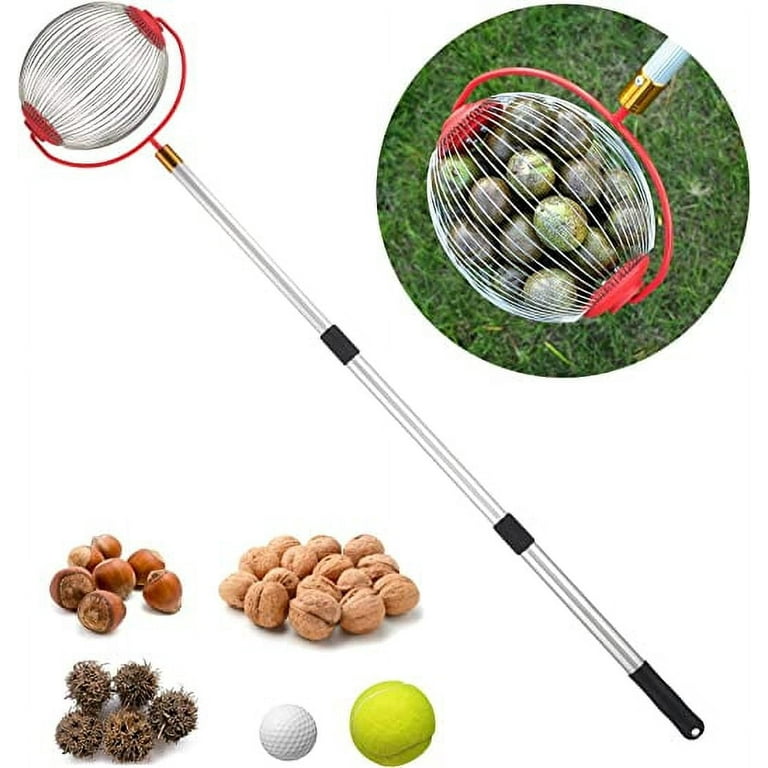The image is an advertisement showcasing a specialized tool designed for picking up various small objects from the ground, particularly round ones. The tool consists of a long, metal pole resembling a broomstick, with a black handle on one end and a wired, oval-shaped catcher on the other end. The catcher features a red ring around its perimeter and two black knobs through its middle. Its wire structure is flexible yet sturdy, enabling it to roll over objects and collect them inside the catcher. In the top right corner of the image, the tool is depicted in use, holding several green round objects against a backdrop of green grass. Below the tool, on the left side of the image, there are separate piles of acorns, walnuts, brambles, a tennis ball, and a golf ball, illustrating the variety of items the tool can effectively pick up. This tool is commonly used on golf courses and other areas where picking up small, round objects from the ground is needed, providing a convenient solution that eliminates the need for bending over.